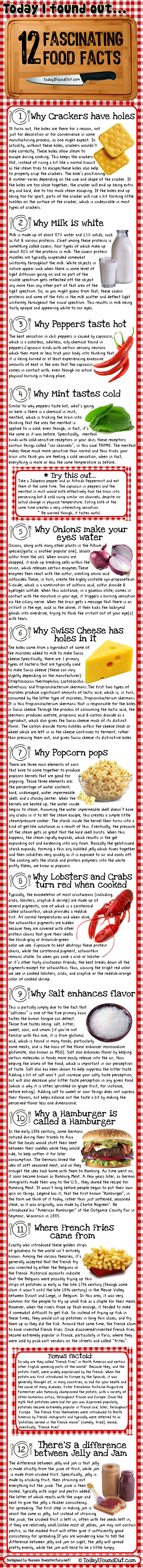The image is a detailed pamphlet titled "12 Fascinating Food Facts," with the title prominently displayed in black capital letters along the top, placed on what resembles a wooden ruler. The pamphlet is divided into twelve sections, each numbered and featuring a title, a photograph of the related food item, and a brief paragraph of information. The paragraphs are written in very small print, making them difficult to read, but the titles of each fact are clearly visible. Here is a detailed description of each fact along with its corresponding image:

1. **Why crackers have holes**: An image of two crackers.
2. **Why milk is white**: A picture of milk in a container.
3. **Why peppers taste hot**: A picture of three chili peppers.
4. **Why mint tastes cold**: An image of several pieces of mint.
5. **Why onions make your eyes water**: A photo of a chopped red onion.
6. **Why Swiss cheese has holes**: A triangular piece of Swiss cheese.
7. **Why popcorn pops**: An image of a bowl of popcorn.
8. **Why lobsters and crabs turn red when cooking**: A picture of a red lobster.
9. **Why salt has a flavor**: An image showing salt on a silver plate.
10. **Why a hamburger is called a hamburger**: A photo of a fully dressed hamburger with lettuce, tomato, and other toppings.
11. **Where french fries come from**: A plate of french fries.
12. **The difference between jelly and jam**: Two jars containing jelly and jam, with the jelly visible next to the containers.

Each section provides intriguing insights into common questions about food, accompanied by visually appealing and relevant images.